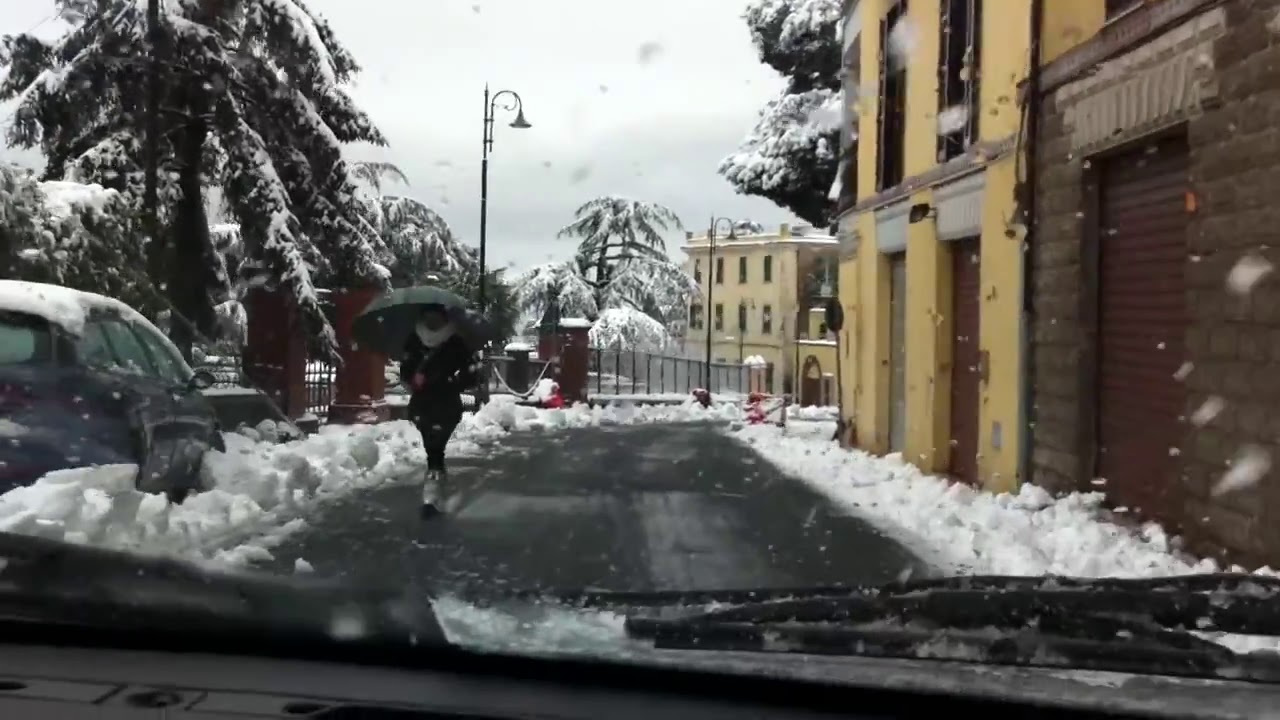A dashcam image captures a snowy winter scene from inside a car. The foreground features the car's black dashboard, windshield wipers, and some ice and water droplets on the window. The road ahead, recently plowed, reveals black asphalt flanked by clumps of freshly fallen snow. On the left side of the road, a blue car, marked with snow on its roof, is parked, while a large silver fence with posts and big evergreen trees covered in snow lines the sidewalk. A person, dressed in a black coat, black trousers, and a white scarf, walks towards the vehicle, clutching a black umbrella and keeping one hand in their pocket.

Beyond the immediate roadside, the background consists of a mix of yellow and beige buildings with black-outlined windows, depicting a European style. One notable building has a brown door and a gray door, with snow-capped trees and a light post nearby. The sky appears white, indicating active snowfall, and additional buildings and a dark structure with a black gate can be seen in the far distance. The image encapsulates a tranquil urban winter scene, highlighting the stark contrast between the dark, wet road and the snow-covered surroundings.